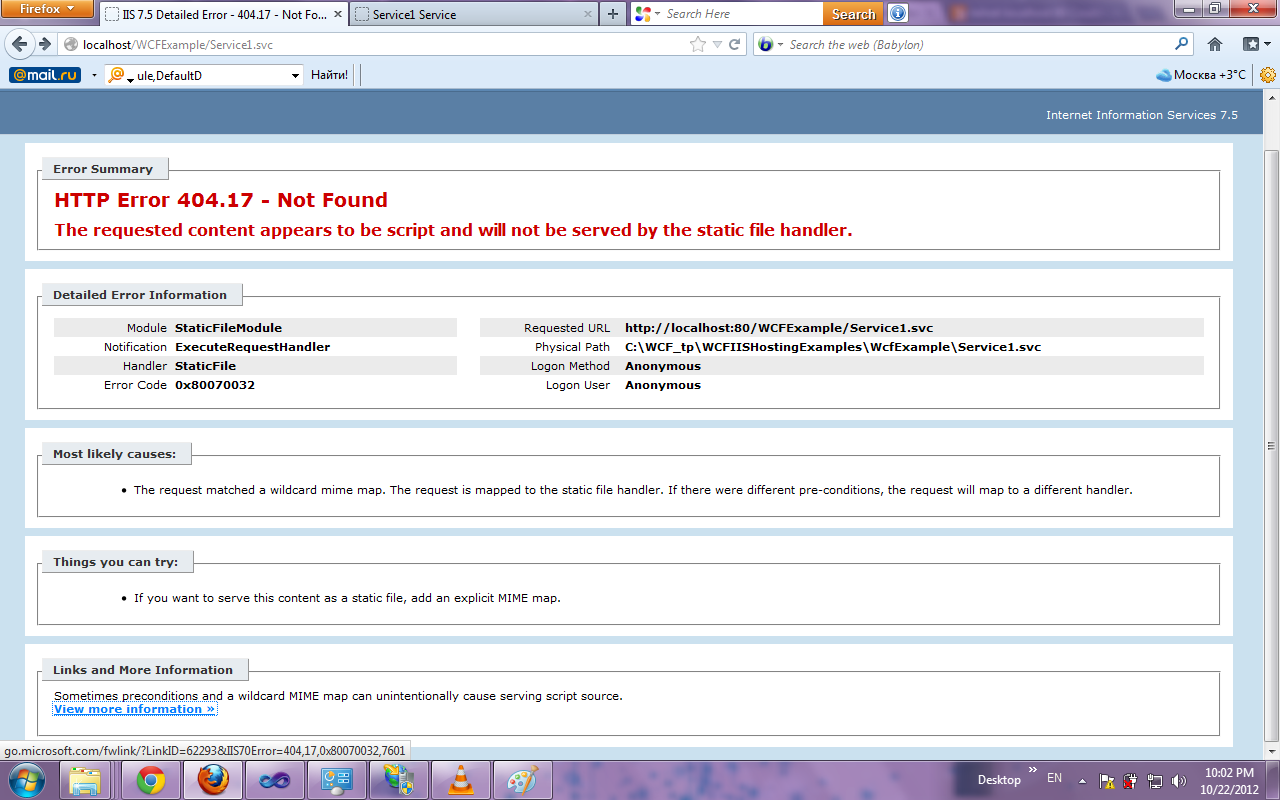The image is a screenshot of a web page displayed in landscape orientation. At the top of the browser, there are multiple open tabs, including a search box that features a Microsoft logo, suggesting it might be Microsoft Edge or possibly an older version of Internet Explorer. Adjacent to the tabs is a long address bar displaying "localhost," followed by an option to "search the web."

The web page features a pale blue border on the left and right edges, as well as across the top. Directly beneath this blue border is a dark blue horizontal band that spans the width of the page, showcasing the text "Internet Information Services" in white.

Below this band, the page is divided into several white information boxes, starting with one that contains a red error message: "HTTP Error 404.17 - Not Found. The requested content appears to be script and will not be served by the static file handler." Just above this message is a gray rectangle labeled "Error Summary."

The next white box, almost stretching the full width of the screen except for the light blue borders, is titled "Detailed Error Information." It provides specifics such as "Module," "Notification," "Error Code," "Requested URL," "Physical Path," and "Login Method."

Following this section, another white box is labeled "Most Likely Causes," outlining potential reasons such as "The request matched a wildcard MIME type" and "The request is mapped to the static file handler."

Below it, a section named "Things You Can Try" offers solutions, one of which suggests adding an explicit MIME mapping if the content is intended to be served as a static file.

Finally, the last white text box is titled "Links and More Information," offering additional links for further details.

At the bottom of the page, a purple band features an array of colorful navigational buttons, including icons representing Microsoft, a file folder, Google, Firefox, and MS Paint's palette program. Also present is an icon resembling a traffic cone, potentially indicating a website builder, as well as a few other icons that are not easily recognizable. One of the links partially visible appears to read "go.microsoft.com."